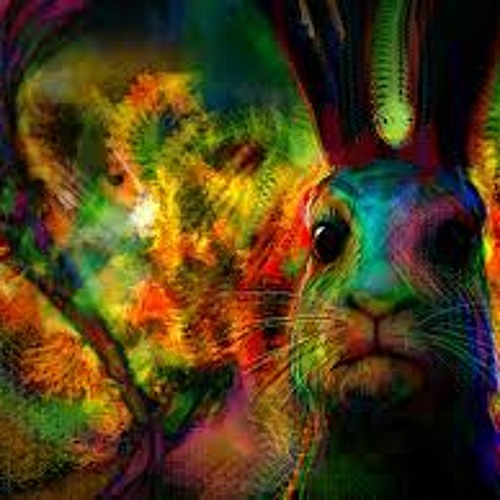In this square, slightly blurry and psychedelic image, we see vibrant, multicolored artwork that appears to be computer-generated. The focal point on the right side is a large rabbit staring directly at us with oversized, dark black eyes. The rabbit’s fur is a tie-dye blend of neon and dark hues, including green, yellow, orange, pink, blue, and purple. Its tall ears, located at the top right corner, are dark red with hints of purple. The rabbit’s face exhibits a kaleidoscope of colors: the right side is blue and pink, the nose is green and yellow, and white whiskers extend in both directions. The background, in contrast, is a blurred, swirling mix of greens, yellows, oranges, reds, purples, and browns, contributing to the image's overall trippy, psychedelic feel. The left side of the image showcases a predominantly purple swirl mixed with green, flowing from the upper left corner to the bottom. There is no discernible text within the image.